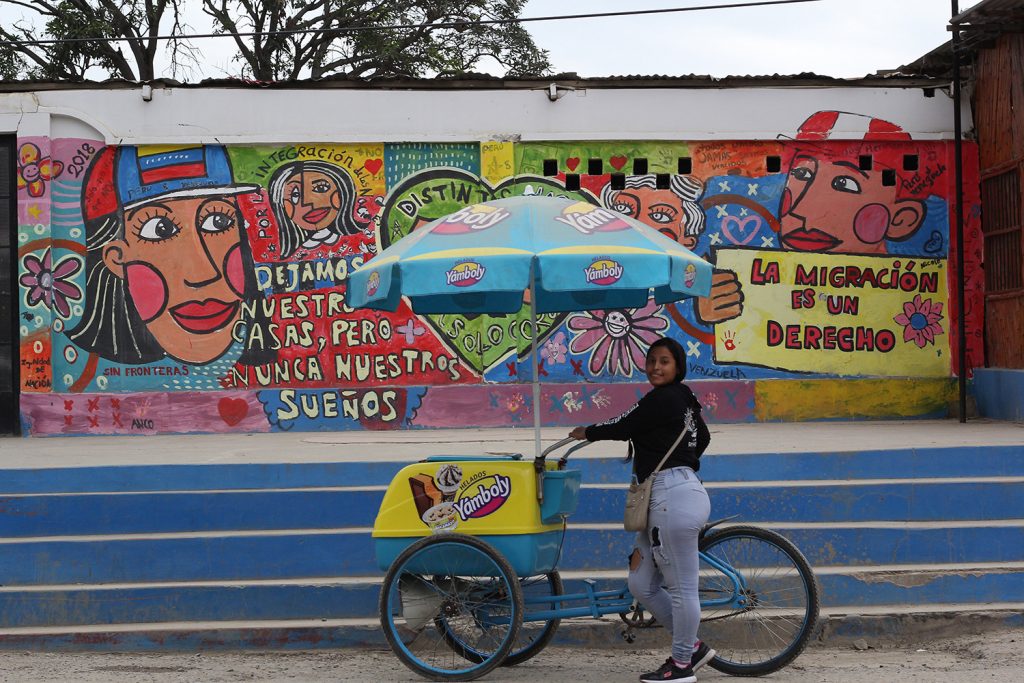The image captures a vibrant scene featuring a dark-skinned woman standing next to a unique blue tricycle, which serves as her mobile vending cart. The tricycle is equipped with an umbrella and a blue-and-yellow plastic container that prominently displays the brand name "Yamboli," indicating she is selling frozen treats such as ice cream and sundaes. The woman, dressed in a black long-sleeve shirt, gray pants, and black shoes, smiles warmly at the camera. 

She is positioned in the center of the image, which is framed as a wide vertical rectangle. The background reveals a colorful, intricately painted wall adorned with a mural that includes various faces—some resembling Aztec figures—and vivid elements like flowers. Spanish words are written on the mural, including a man on the right holding a yellow sign with red text that reads, "La migración es un derecho." In front of the mural is a white concrete platform that contrasts with the gray ground on which she stands. Leading up to the mural are striking blue stairs, and above the building, trees and a patch of sky can be seen, adding an extra layer of depth to the image. This lively street scene likely takes place in Mexico, as suggested by the Spanish text and cultural motifs.